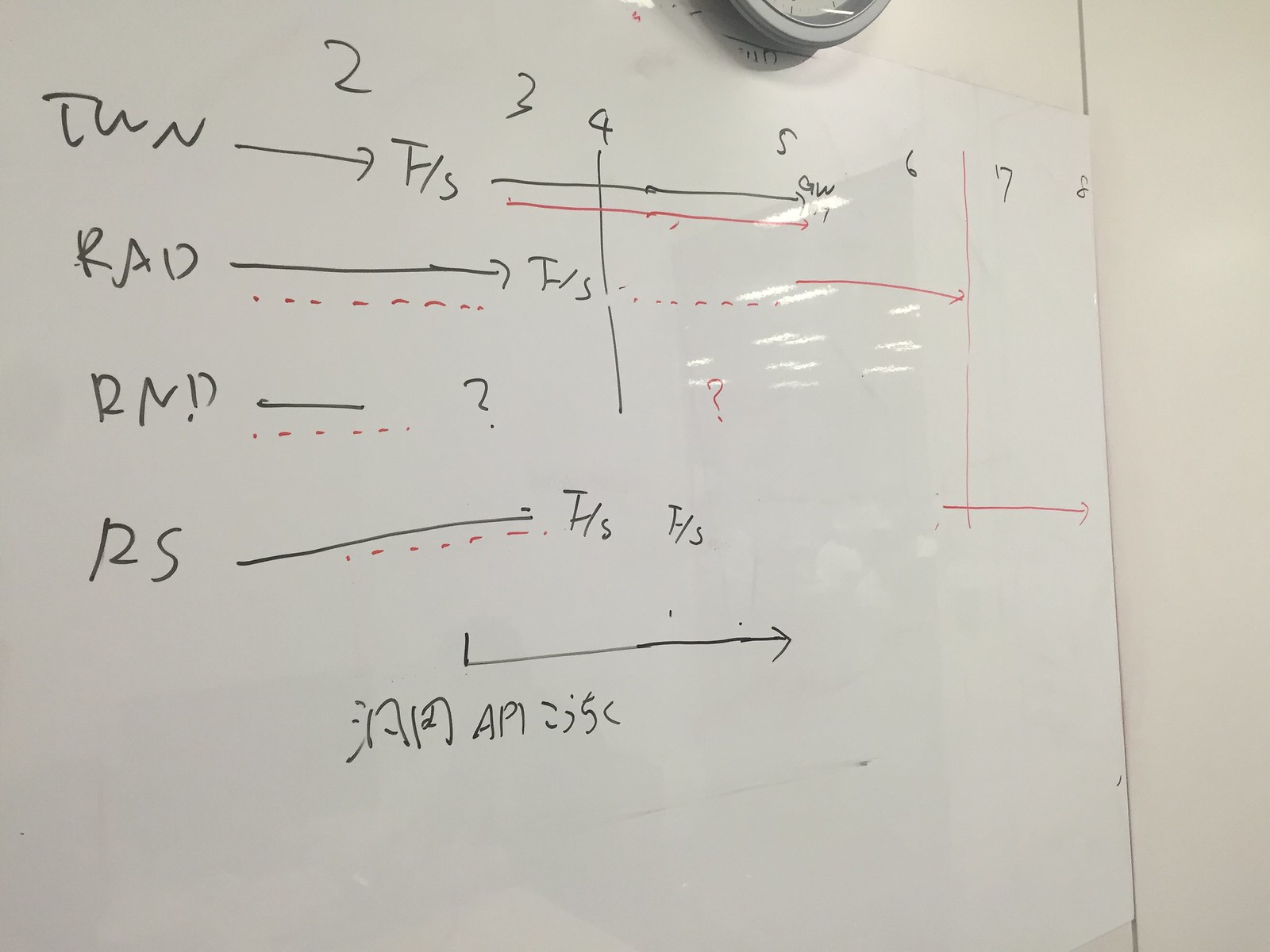This photograph captures a whiteboard mounted on the wall in what appears to be a classroom, lecture hall, or workspace. The whiteboard is plain and unframed, providing a functional surface for writing. Above the whiteboard, the bottom edge of a clock with a silver plastic frame is visible, though the numbers and hands cannot be seen.

The whiteboard is filled with numerous black dry erase marker inscriptions. Across the top of the board, the numbers 1 through 8 are written in a sequence. Below these numbers are an array of black abbreviations and words that are largely indecipherable. 

Some notable markings include:
- The letters "T-U-N" with an arrow pointing to "F/S," followed by a long arrow extending under the number 5.
- The abbreviation "G-W" appearing next. 
- "R-A-D" connected via a long arrow to "F/S," and then a red arrow points to a vertical line located between the numbers 6 and 7.
- "R-N-D" with a shorter arrow leading to a question mark, flanked by a red question mark located under the space between the numbers 4 and 5.
- Below, "R-S" connects through a longer arrow to "F/S," found under the number 3, and another "F/S" just to the right of the number 4.

The lower portion of the whiteboard features additional writing that resembles Chinese characters or another form of Asian script, interspersed with the Latin acronym "A-P-I."

The whiteboard's densely packed content suggests it serves as a dynamic tool for conveying complex information, possibly related to a brainstorming session, class lecture, or project planning.